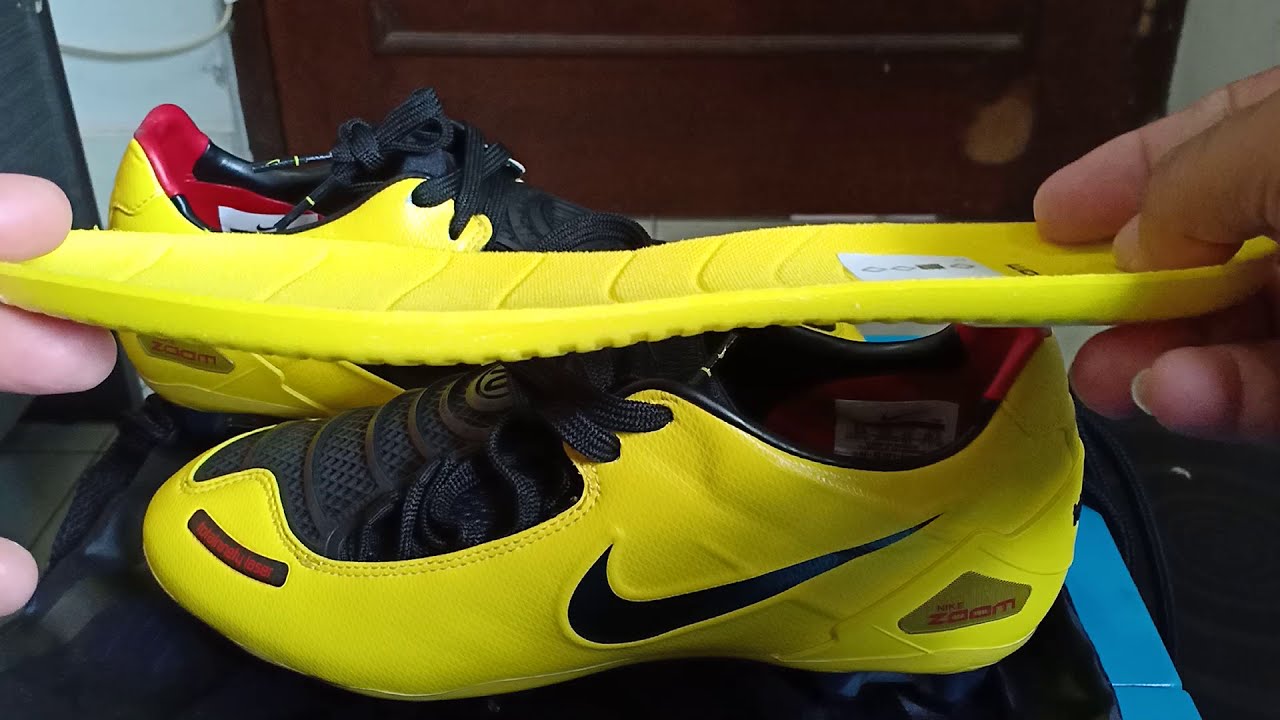The photograph captures a pair of bright yellow Nike sports shoes positioned on a flat surface, with the shoe in the foreground oriented so that its toe points to the left and its heel to the right. The partner shoe is positioned behind it, facing the opposite direction. Both shoes feature black laces and a black tongue, with "Zoom" marked in red text at the heel. The interior of the shoes is a combination of black and red. Above the shoes, a person is holding a matching yellow insole, identified by visible white fingers on both sides—left fingers gripping the edge while the right hands firmly clasp it between fingers. The setting appears to include a white wall and a wooden door in the background, adding context to the scene.